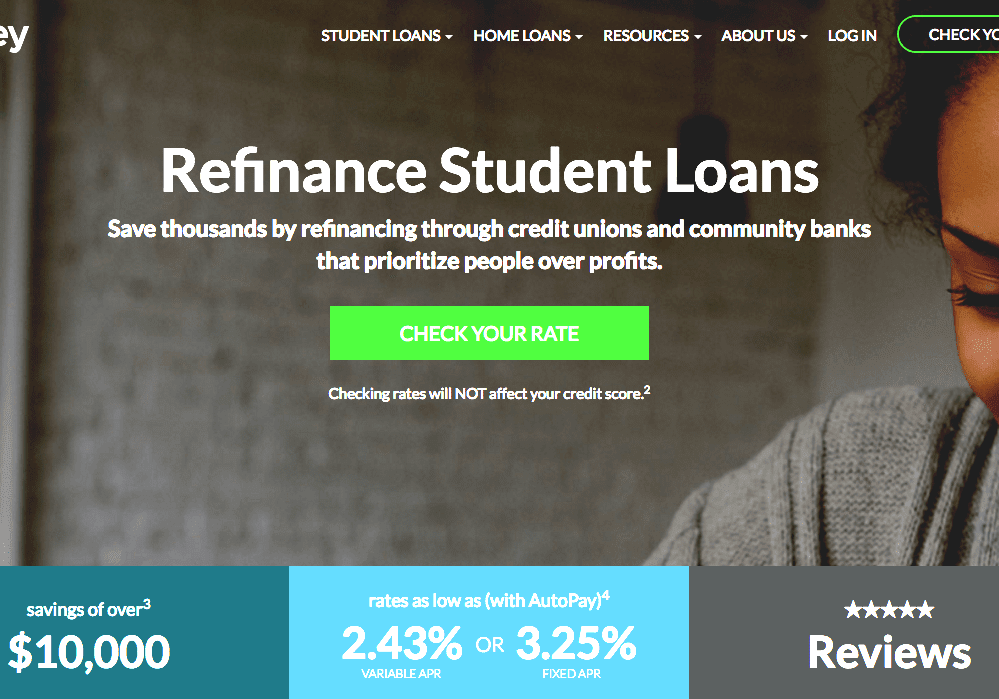The image is a partial screenshot from a website, missing significant portions on the left and right sides. The complete website name is not visible, with only the white text "EY" discernible. The background features a photograph of a woman, displaying just the right side of her face. She has dark hair and light brown skin and is wearing a gray sweater.

At the center of the image, large white text promotes refinancing student loans, highlighting that individuals can save thousands by refinancing through credit unions and community banks that prioritize people over profits. Below this text, there is a prominent green button with white text reading "Check Your Rate," followed by an assurance in smaller white text that "Checking rates will not affect your credit score."

Beneath this, several colored boxes provide additional details. A blue box announces potential savings of over $10,000, another lighter blue box advertises rates as low as 2.43% or 3.25% with auto pay, and a gray box contains customer reviews.